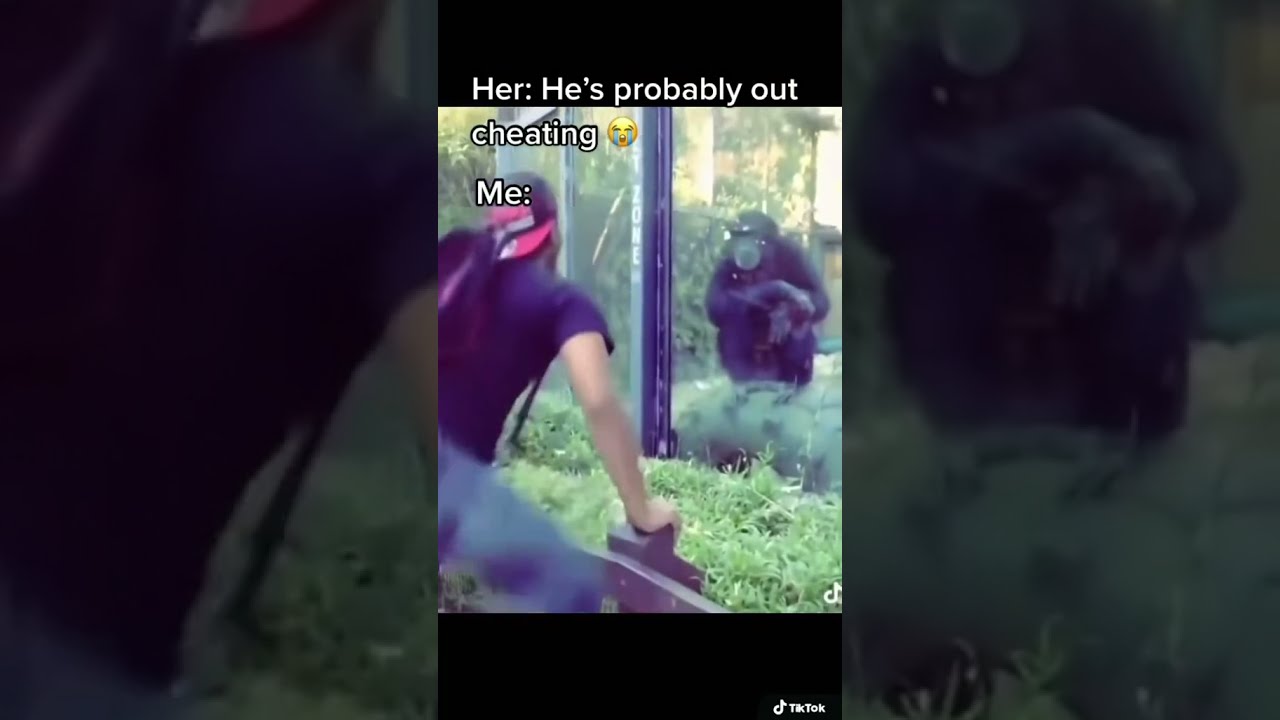This is a humorous TikTok screenshot featuring an image within an image. The main picture, lightly colored and centrally positioned, occupies about a third of the screen against a darker, slightly opaque background version of the same scene. At the top, text reads, "Her: He's probably out cheating," accompanied by a crying emoji, while below it, the caption says, "Me," suggesting a contrast. The central image shows a black man in a black shirt, jeans, and a red and black backwards hat, leaning over a fence barrier at the zoo. He is peering through a glass window at a squatting chimpanzee, who glares back with its arms crossed over its knees. The scene includes grass and bushes between the wooden barrier and the window, with the word "zone" visible on the post. The TikTok logo is displayed at the bottom of the screen, indicating that this is part of a humorous TikTok post.